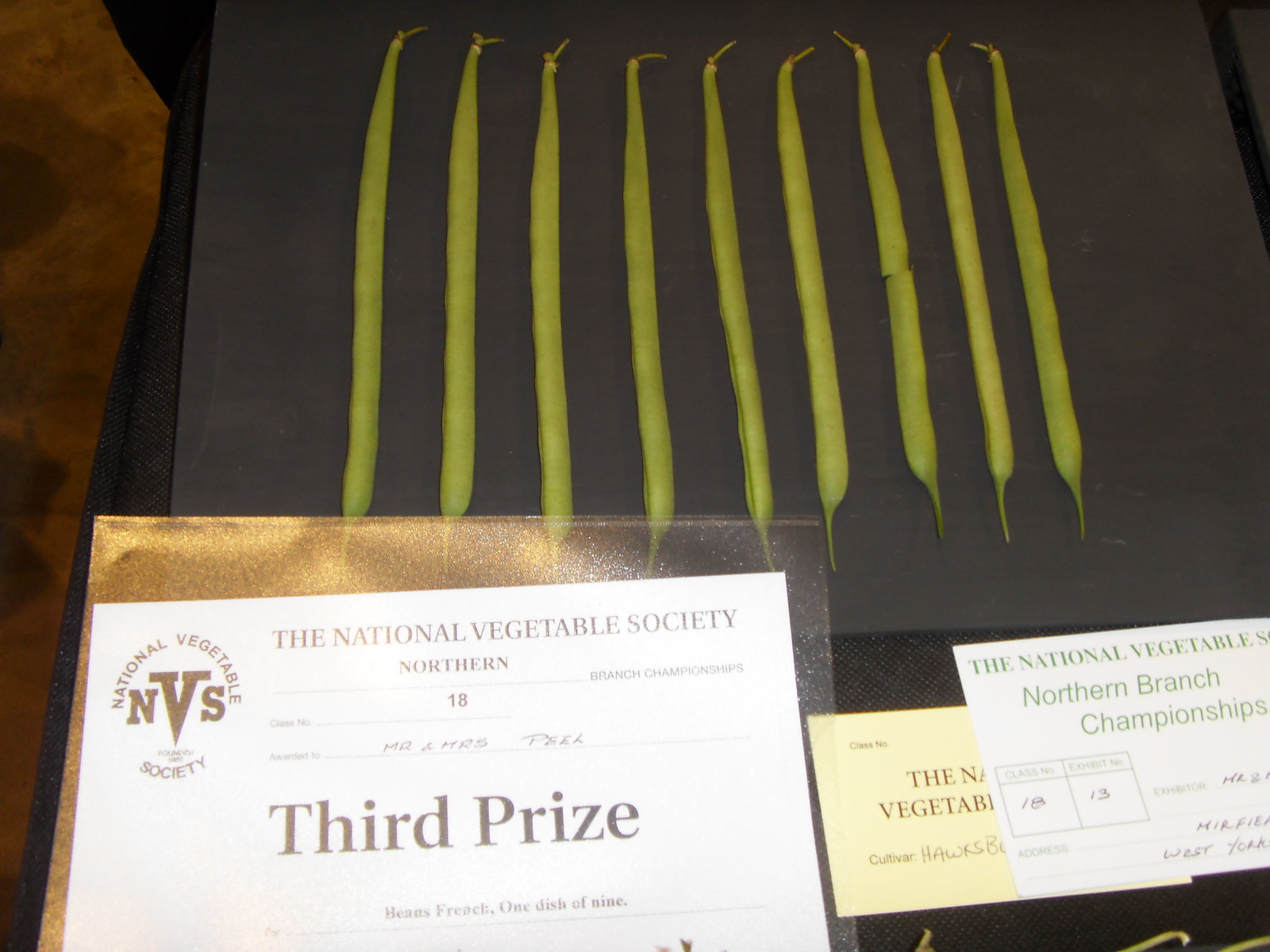The image depicts an award event from a vegetable competition, specifically showcasing green beans. The beans are arranged vertically on a dark surface, which appears to be black material paper. Beneath the beans is a white paper in a plastic protector, which reads: "The National Vegetable Society Northern Branch Championship, Class Number 18, Mr. and Mrs. Pill, Third Prize, Beans French, One Dish of Nine." Next to the third prize award is another card bearing the text: "The National Vegetable Society Northern Branch Class Number 18, Exhibit 13." The prominent focus of the image is the neatly displayed green beans and accompanying awards, highlighting their recognition in this prestigious vegetable contest.